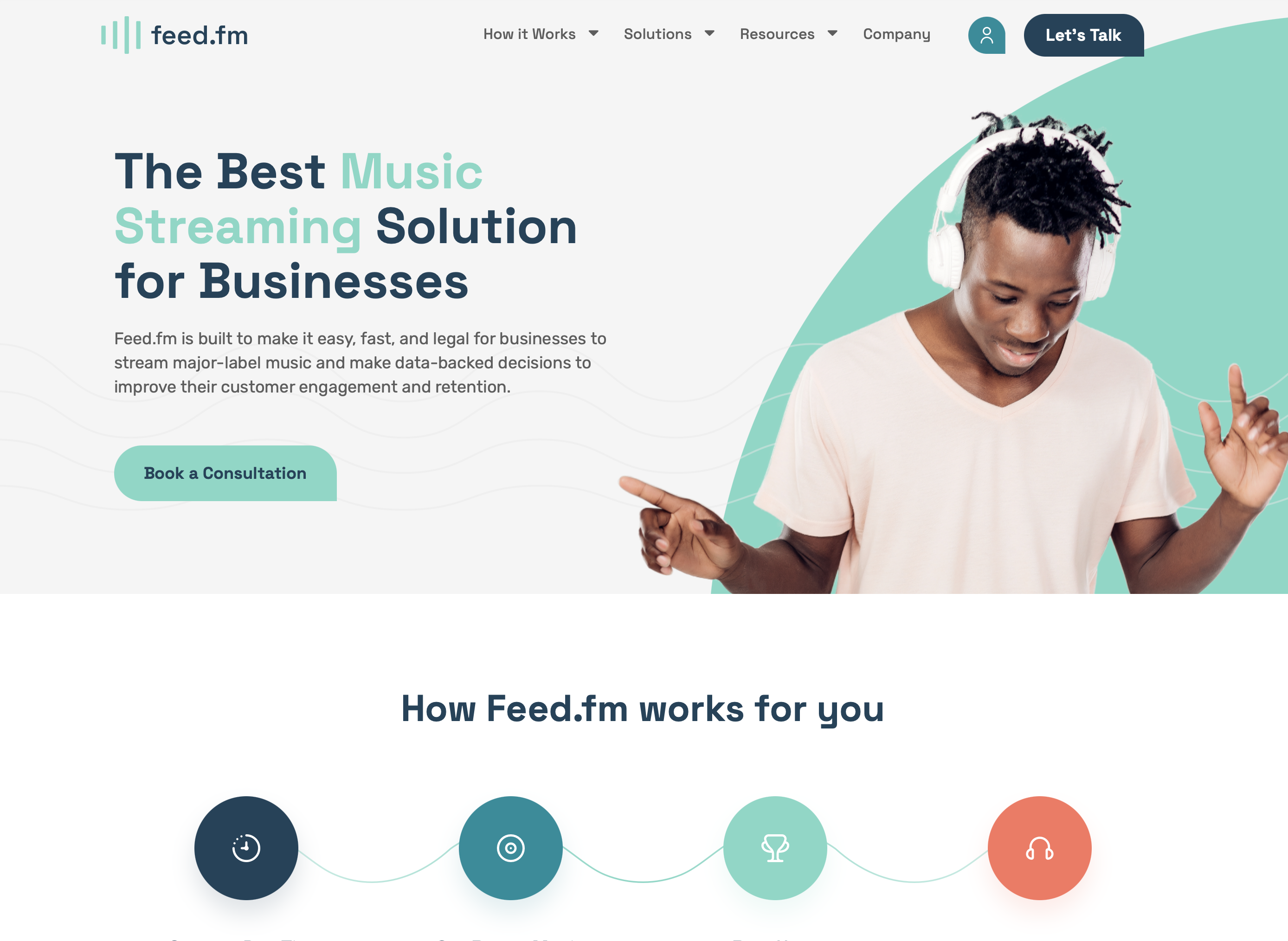The advertisement for Feed.fm features a vibrant design to draw attention to its offerings. At the center of the image is a prominent white box. Within this box, there is a striking aqua half-circle that frames a lively figure. This person, sporting white headphones and a cream-colored shirt, is captured mid-dance, embodying the joy and energy of music.

At the top of the advertisement, there are navigation tabs in navy blue: "How It Works," "Solutions," "Resources," "Company," and "Let's Talk." Below these tabs, a bold headline reads, "The Best Music Streaming Solution for Businesses," with the phrase "music streaming" highlighted in aqua, contrasting against the rest of the text in navy blue.

A concise description follows: "Feed.fm is built to make it easy, fast, and legal for businesses to stream major label music and make data-backed decisions to improve their customer engagement and retention." This text underscores the platform's value proposition.

Towards the bottom, an aqua box with navy blue writing invites readers to "Book a Consultation." Beneath this call-to-action is a section titled "How Feed.fm Works for You." This part features a visual flowchart starting with a blue circle containing three-quarters of a circle with a V shape, connected by a string to a teal circle resembling a CD. The string continues to a green circle with a trophy icon and finally leads to an orange circle with headphones, illustrating the streamlined process of using Feed.fm.

Overall, this advertisement effectively communicates the utility and advantages of Feed.fm's music streaming solution for businesses.